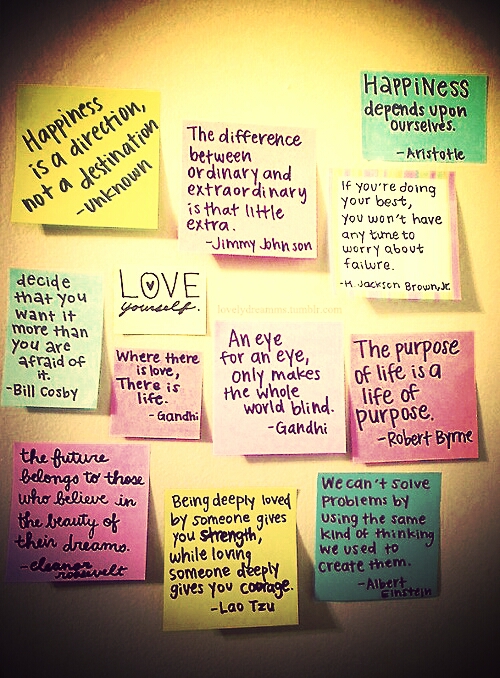This photograph showcases a collection of colorful sticky notes meticulously arranged on a tan wall, with an intriguing dark vignette around the edges that directs focus to the notes themselves. Each sticky note, in hues of yellow, green, white, and pink, features a positive and motivational quote. In the top left corner, a yellow sticky note displays the quote, "Happiness is a direction, not a destination," attributed to an unknown author. Adjacent to the right, a pink sticky note states, "The difference between ordinary and extraordinary is that little extra," by Jimmy Johnson. Further to the right, a green sticky note reads, "Happiness depends upon ourselves," by Aristotle. The bottom left corner features a quote by Eleanor Roosevelt on a pink sticky note, which says, "The future belongs to those who believe in the beauty of their dreams." To its right, another sticky note, possibly green, carries Lao Tzu's wise words: "Being deeply loved by someone gives you strength, while loving someone deeply gives you courage." Finally, in the bottom right corner, a quote by Albert Einstein on yet another note reminds us, "We can't solve problems by using the same kind of thinking we used to create them." Each quote is carefully inscribed, adding to the overall inspirational theme conveyed through this vibrant display.